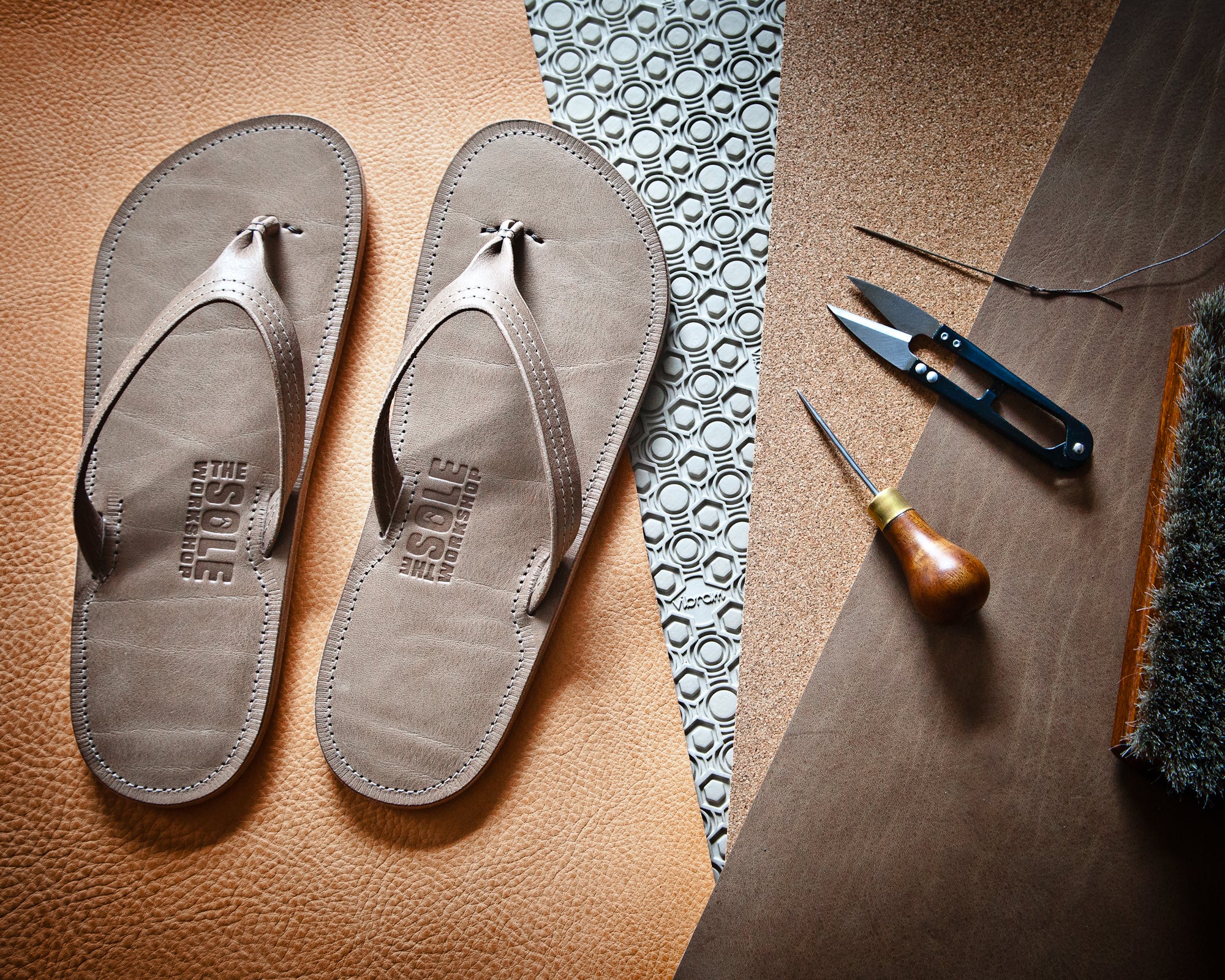In a professionally lit and clear image, a pair of brown leather flip-flops rests on a strip of tan leather. The soles of the flip-flops, which bear the embossed text "The Sole Workshop," sit centrally, suggesting a promotional photograph for a sandal company. To the right of the flip-flops, a selection of leather-cutting tools is arranged on a textured silicone mat, which features circular and hexagonal patterns. Among the tools are a pair of sharp, black-handled shears, a wooden-handled chiseling tool, and a small needle on a wire that resembles a twist tie. Additionally, a vertical long brush is visible peeking in from the right edge of the image. The combination of these elements indicates a workshop setting where the sandals might be crafted.